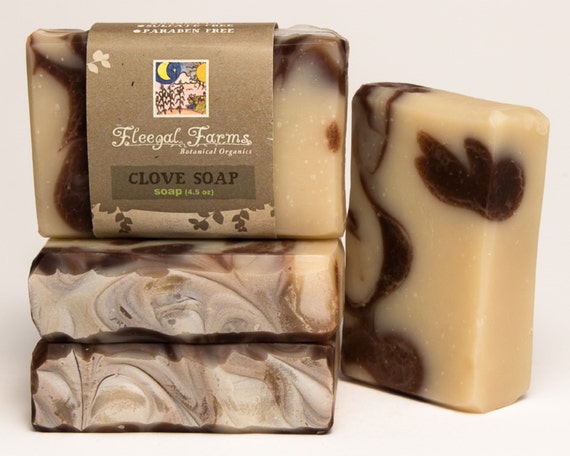This highly detailed photograph presents a set of four artisanal bars of soap displayed thoughtfully against a white background. Each bar exhibits a cream-colored base intricately marbled with black swirls, accentuating their handmade appeal. On the uppermost position, a vertical bar of soap prominently showcases its face, adorned with a brown cardboard label detailing the product's natural and organic attributes. The label bears the name "Flegal Farms Botanical Organics," with an illustration of a forest, sun, and moon above the prominently displayed text "Clove Soap." Additionally, it specifies the weight as 4.5 ounces and highlights that the soap is paraben-free and sulfate-free. To the left of this, two bars are neatly stacked in a horizontal arrangement, with a fourth bar positioned vertically beside them to better display the soap's intricate design. This composition suggests not only the handmade quality of the soap but also its potential as a gift set or promotional display, emphasizing natural ingredients and aesthetic craftsmanship.